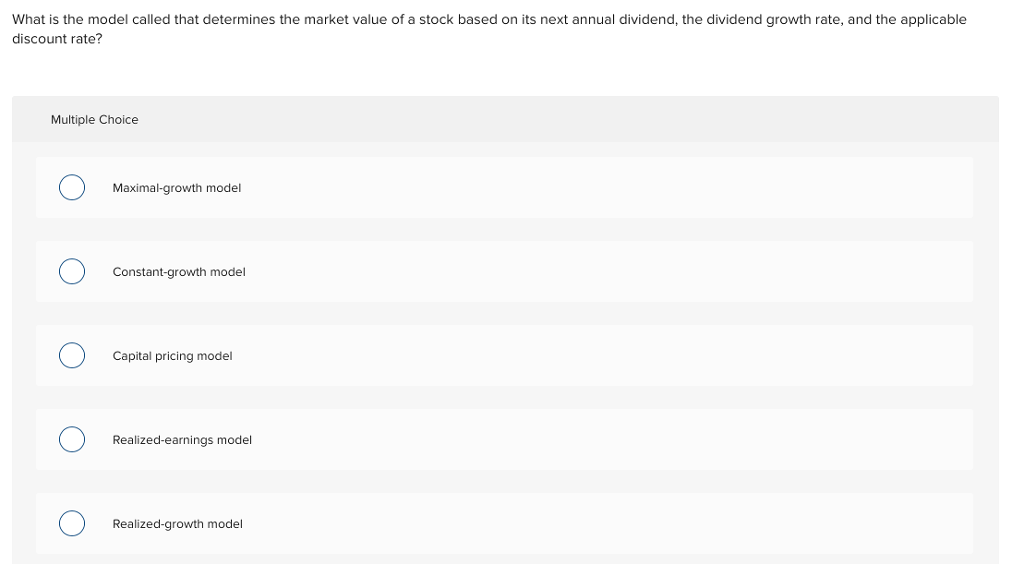In the image, a large rectangular screen displays a multiple-choice question with a light gray background. At the top of the screen, a narrow strip of medium gray, slightly darker than the main background, prominently features the label "Multiple Choice" in small, plain black text using a basic sans-serif font. Below this header, there are five answer options, each presented within a long rectangular strip that has an almost off-white background. 

Each answer option is accompanied by a white circular tick box bordered by dark blue. The answer options are listed in the following order: 

1. Maximal-Growth Model
2. Constant-Growth Model
3. Capital Pricing Model
4. Realized-Earnings Model
5. Realized-Growth Model

The text for each answer is similarly small, plain, and black, using a basic sans-serif font. None of the tick boxes next to the answers have been ticked off, as they appear unmarked by any check marks or highlights. The visual layout suggests this screen is part of a quiz interface, likely for educational purposes or training sessions. The answer sections are roughly double the size of the narrow header strip above.